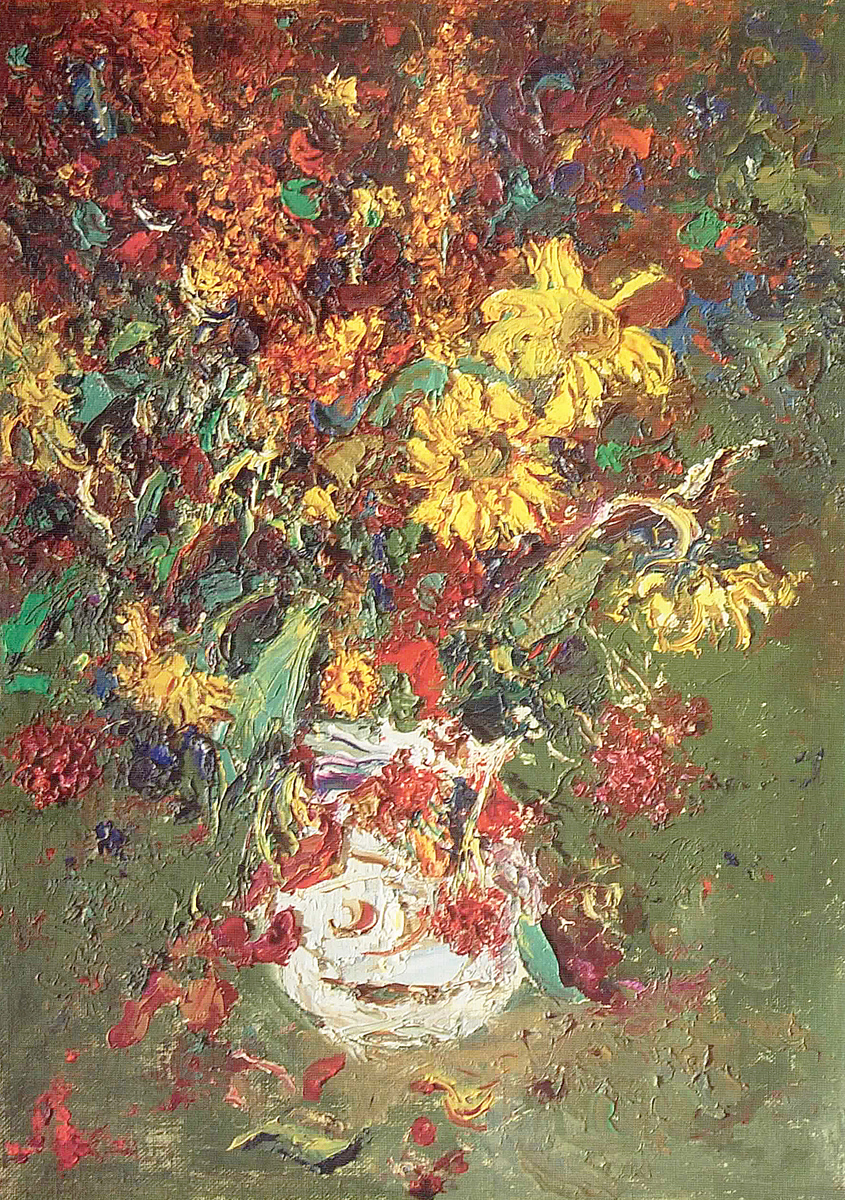The image is an abstract painting that evokes a floral still life, characterized by thick, textured oil paints. Dominated by a green background, the composition hints at a bouquet of fall-colored flowers, with bright yellows, muted oranges, and reds creating a vibrant yet subdued palette. Pops of blues and turquoises add depth and contrast. Among the abstract patterns, one can discern the suggestion of a white vase and sunflower-like shapes, especially on the right side, with the left side blending into an amalgamation of flower-like forms. The artist appears to have utilized a spatula and possibly finger painting techniques, blending colors and textures masterfully to create an impressionistic vision that emphasizes both color and form.